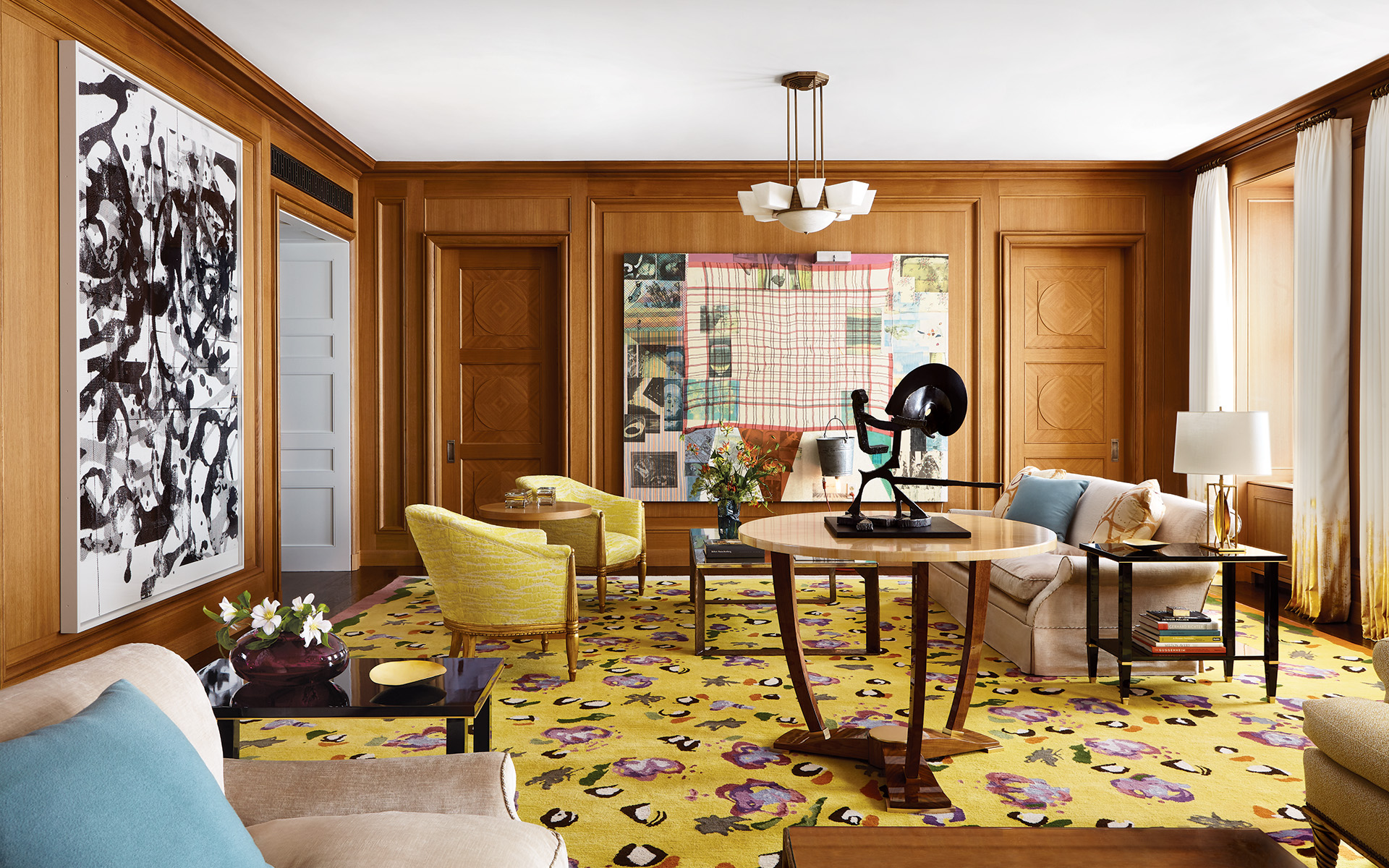The image depicts a brightly lit, eclectic living room that exhibits a mix of modern and abstract decor elements. At the top, the ceiling is stark white, providing a clean background that emphasizes other room details. Dangling from a brown circular feature are brown lines with white, angular, paper-like objects, adding an artistic, surreal touch. The room houses a circular wooden table in the center adorned with a peculiar, abstract sculpture reminiscent of a surrealist gladiator. This table, notably, has only three legs.

To the left of the central table, there are two single yellow chairs with comfortable armrests and back support, positioned around another smaller circular wooden table. On the right side of the room, a beige two-seater couch is adorned with three pillows—one blue and two brown—offering a cozy and inviting seating option.

A yellow rug with an intricate pattern of black, white, purple, and brown hues covers the floor, anchoring the room's vibrant and offbeat aesthetic. Adjacent to the sofa is a larger square wooden table. Mounted on the wooden-paneled wall is a patchwork fabric piece featuring a seemingly random mix of pink, black, white, and brown patches, adding a whimsical touch to the decor.

Further enhancing the room's artistic vibe, a black-and-white canvas painting that looks like a splatter of paint decorates the wall, offering a chaotic contrast to the more structured elements. A white door is visible on the left side of the image, flanked by floor-length curtains, further blending functionality with artistic expression in this captivating and unique living space.